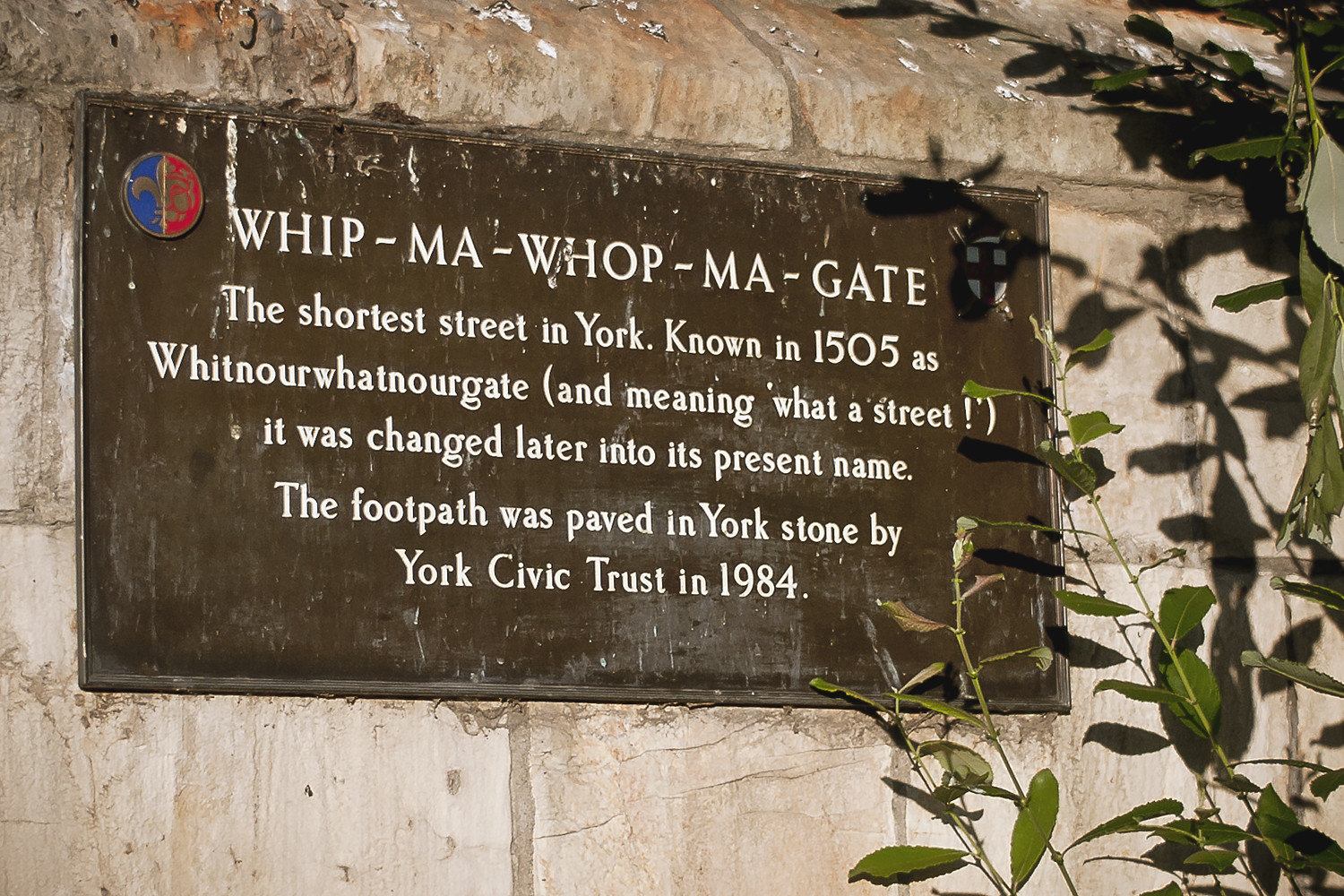The image depicts a dark brown plaque against a wall made of large gray stones, partially obscured by green leaves from nearby branches. The plaque commemorates the Wip-Ma-Wop-Ma Gate, reputedly the shortest street in York, originally known in 1505 as Wip-Nar-Wop-Nar-Gate or Witnawer Watnawer Gate, which means "what a street." This name was later changed to its current form. The text on the plaque is white and in its upper left corner features a fleur-de-lis on a half-blue, half-red circular background. The upper right corner displays a shield with a cross. Additionally, the footpath was paved in Yorkstone by the York Civic Trust in 1984.